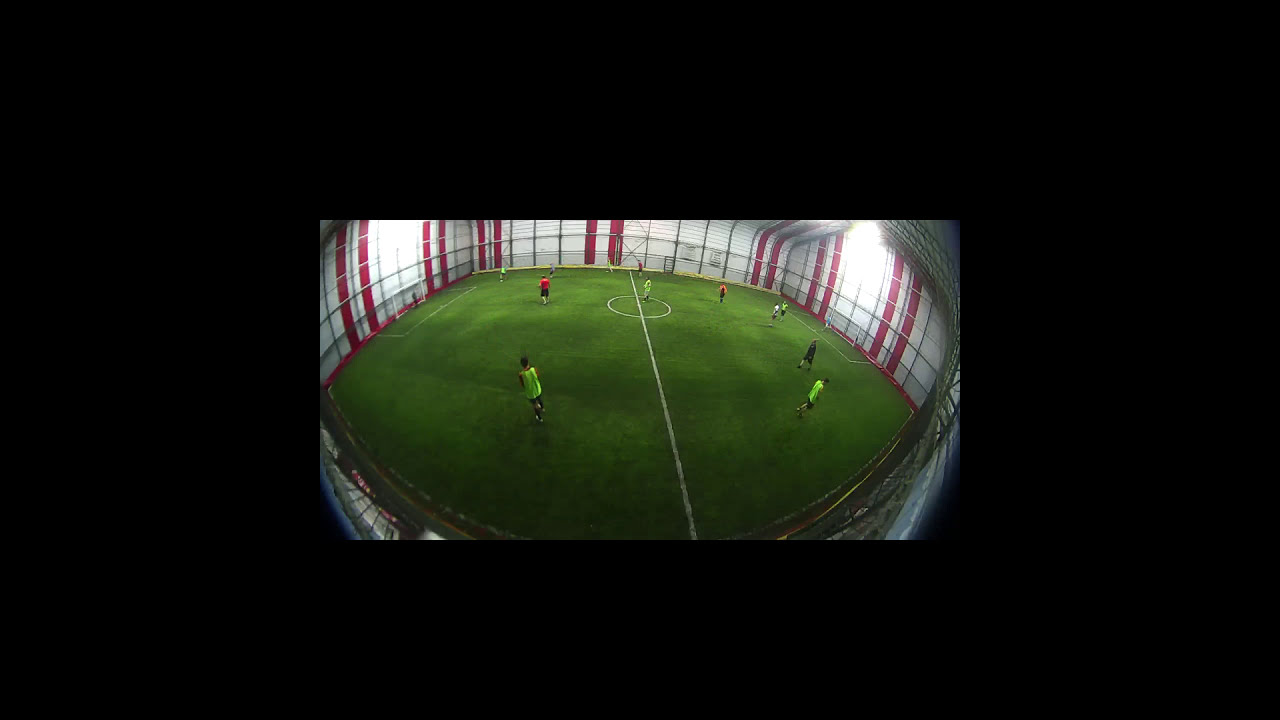The image depicts an intense indoor soccer game unfolding on a rectangular, green turf field that dominates approximately three-fourths of the frame. The turf is adorned with white lines, including one dividing the field in half, and a central circle. Soccer goals are situated against the left and right walls. The walls themselves are predominantly white, decorated with red vertical stripes and red paint along the bottom edges, while the back wall features a yellow border at its base. The soccer players are scattered across the field, with one goalie positioned to the left and another to the right. The athletes are dressed in a variety of jerseys, including light green, black, red, orange, and lime green, suggesting a mix-and-match approach to uniforms. Despite the recreational nature of their attire, the game appears competitive, with the majority of the players concentrated on the right side of the field, where all the action seems to be taking place. There is no text in the image, and it is presented against a plain black background, focusing attention solely on the vivid and dynamic scene within the photograph.